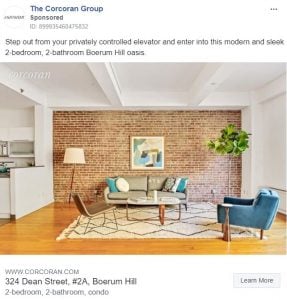This color photo captures a web page displaying a real estate listing, likely for a short-term or vacation rental such as those found on Airbnb or Vrbo. The listing is presented by The Corcoran Group. The description invites potential renters to "step out from your privately controlled elevator and enter into this modern and sleek two-bedroom, two-bath Boerum Hill oasis." 

The living room exudes a contemporary aesthetic with modern chairs, a couch, and a striking brick wall directly facing the camera. A floor lamp and a large artificial tree add to the room's ambiance. The space is adorned with a stylish rug and features a teak or oak-finished floor. To the left, there is a glimpse of a compact, modern kitchen. 

The bottom left corner of the page displays the property's address along with a concise description, accompanied by a "Learn More" button for additional information.